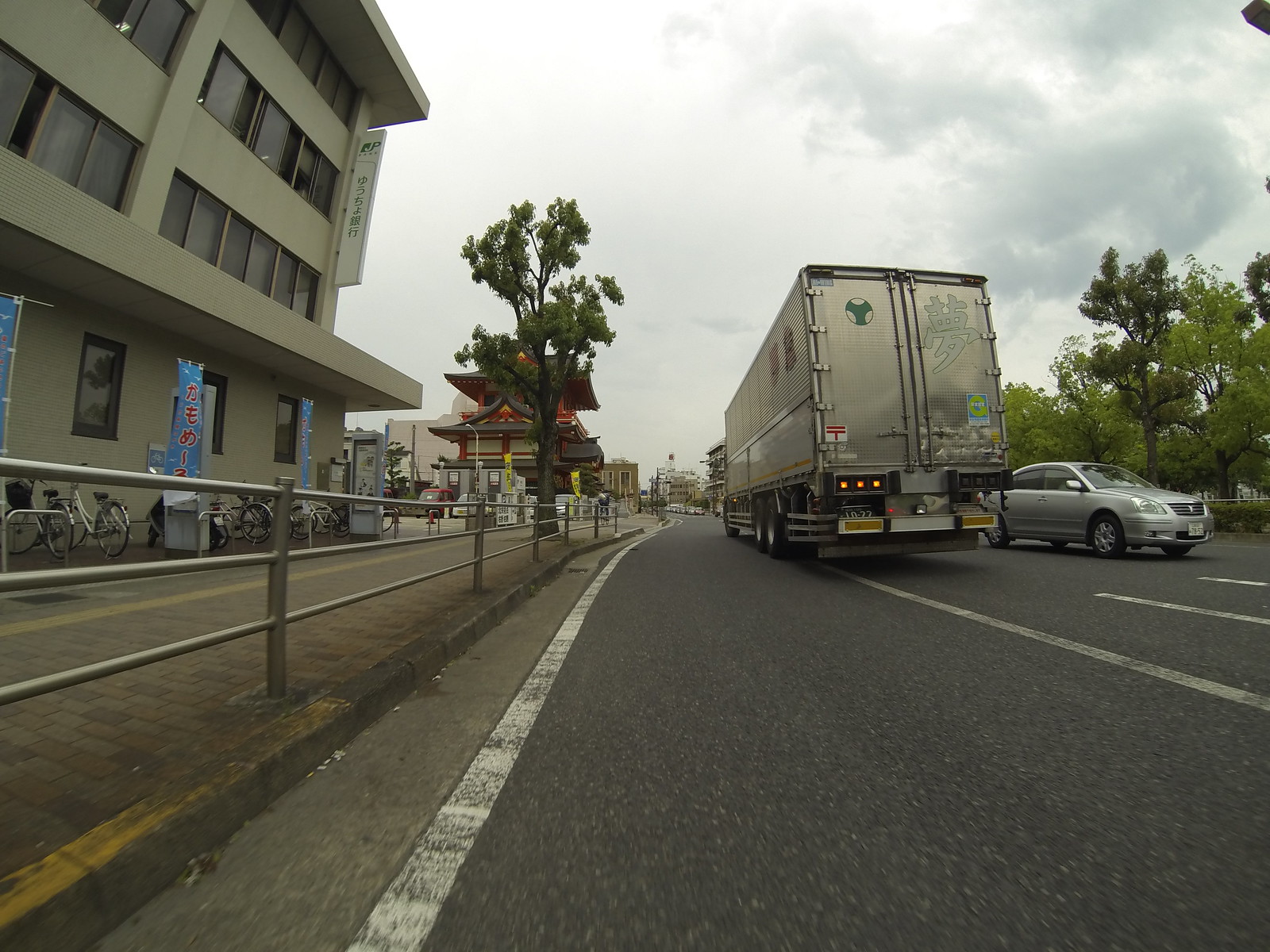In this outdoor city scene, a large 18-wheel truck adorned with a nuclear symbol on one of its back doors is the focal point, moving away from the viewer. A gray sedan is driving in the opposite direction of the truck. The sky above is gray and overcast, with several clouds concentrated in the top right corner. To the left, a cement building stands prominent, with a bicycle rack filled with several bicycles positioned in front of it. The foreground features a brick sidewalk bordered by a metal railing that extends along its length. A single tree is planted on the sidewalk, while the opposite side of the street, across from the gray car, is lined with several more trees.